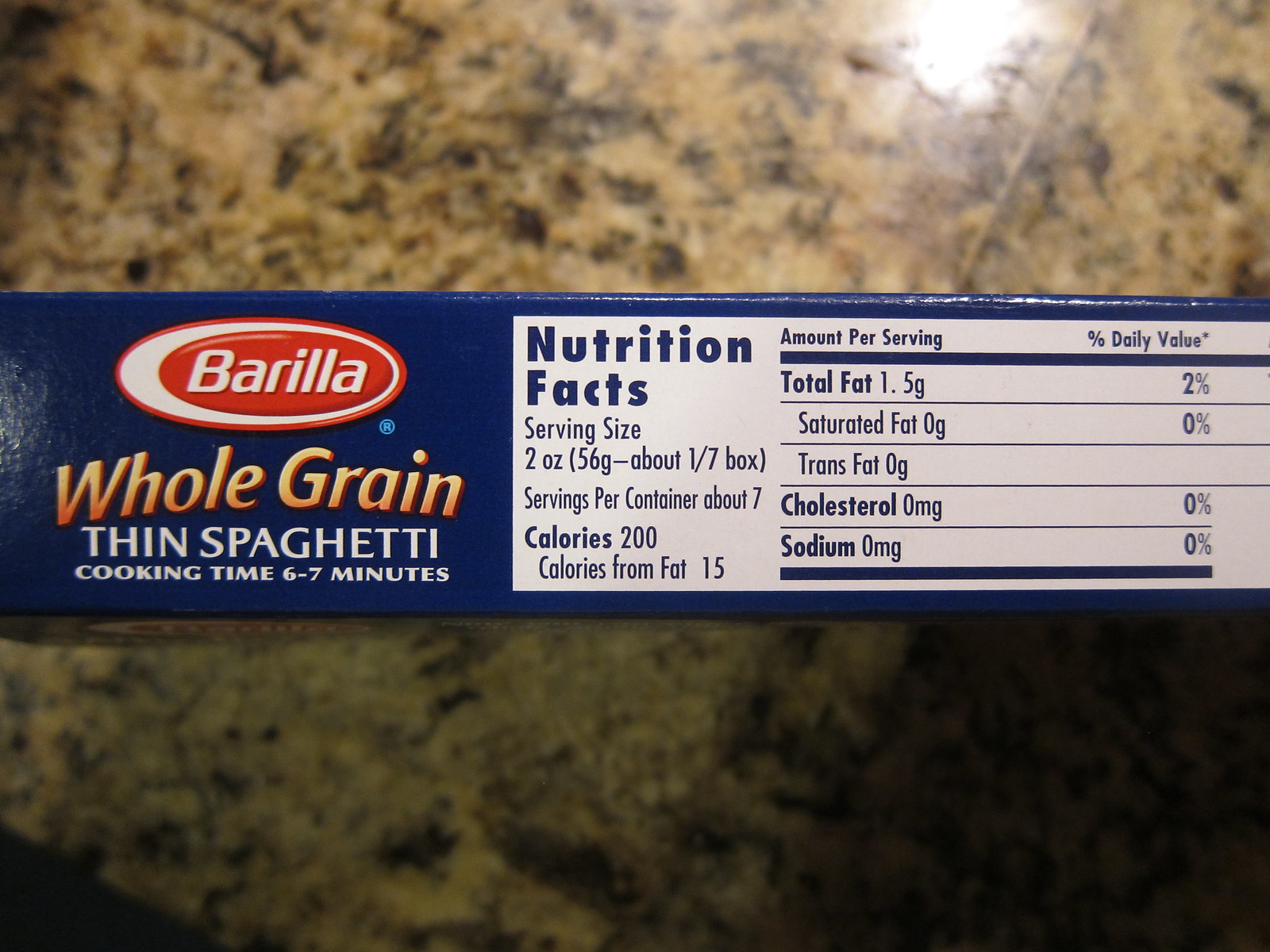The image showcases the side of a rectangular spaghetti package. Dominating the top-left corner is a red oval, centrally featuring the brand name "Brelia." Below the brand name, the package indicates "Whole Grain Thin Spaghetti" and specifies a cooking time of 6-7 minutes. To the right, the nutrition facts table is prominently displayed in white against a dark blue background, detailing values for total fat, saturated fat, trans fat, cholesterol, sodium, calories, and calories from fat. The entire packaging is dark blue in color. In the background, a kitchen counter, colored light brown and black, subtly frames the scene.